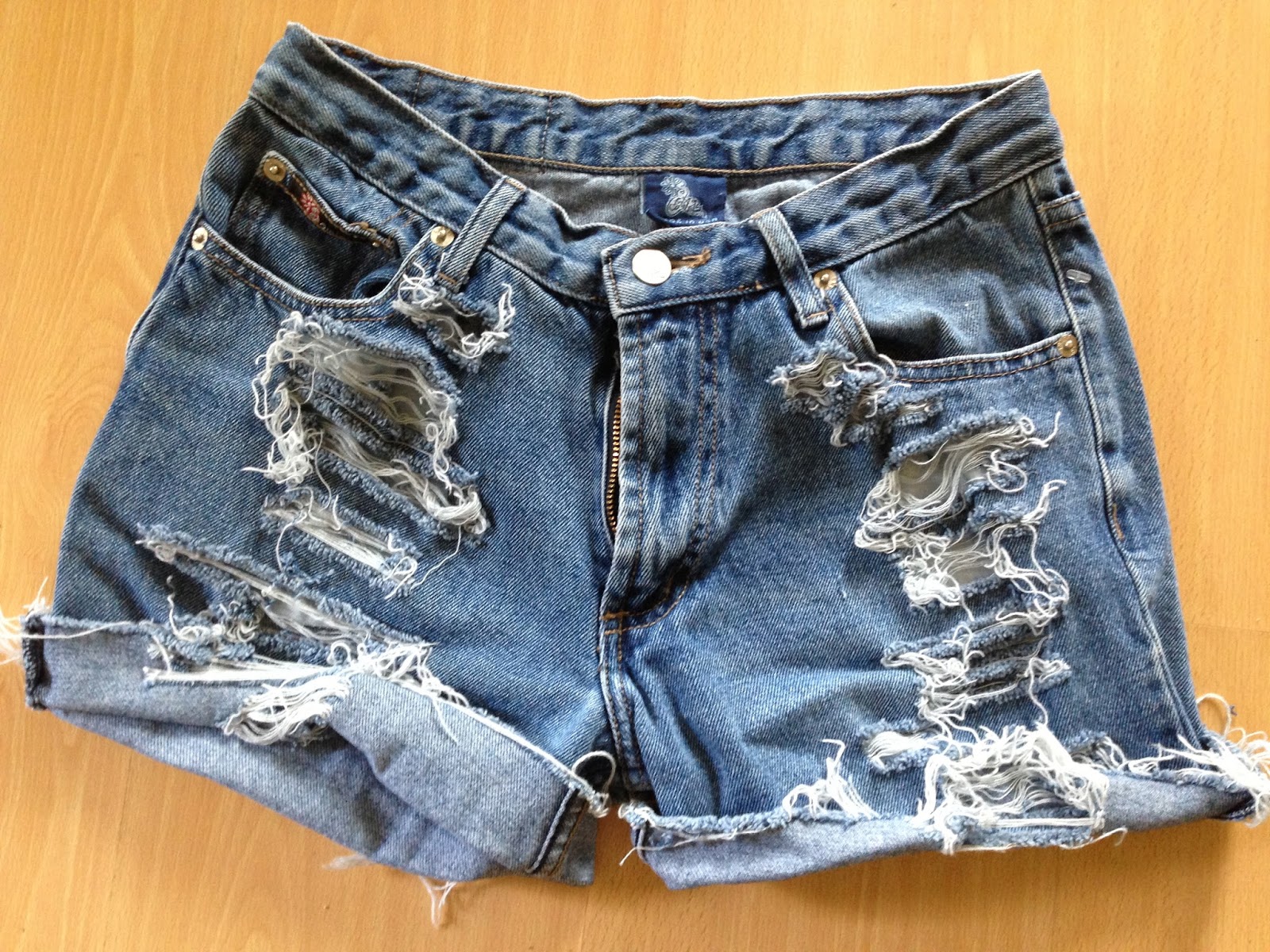This photograph showcases a pair of distressed jean shorts, artfully arranged on a light wood grain background, possibly a floor or table. The stylishly worn shorts feature significant distressing, with frayed fabric and holes prominently on both sides, particularly near the pockets. The bottoms of the shorts are fashionably rolled up, though the left side appears more unraveled than the right. The shorts are buttoned at the top, accompanied by an unzipped zipper and two front pockets. A blue tag with white details is visible, though its text is indiscernible.